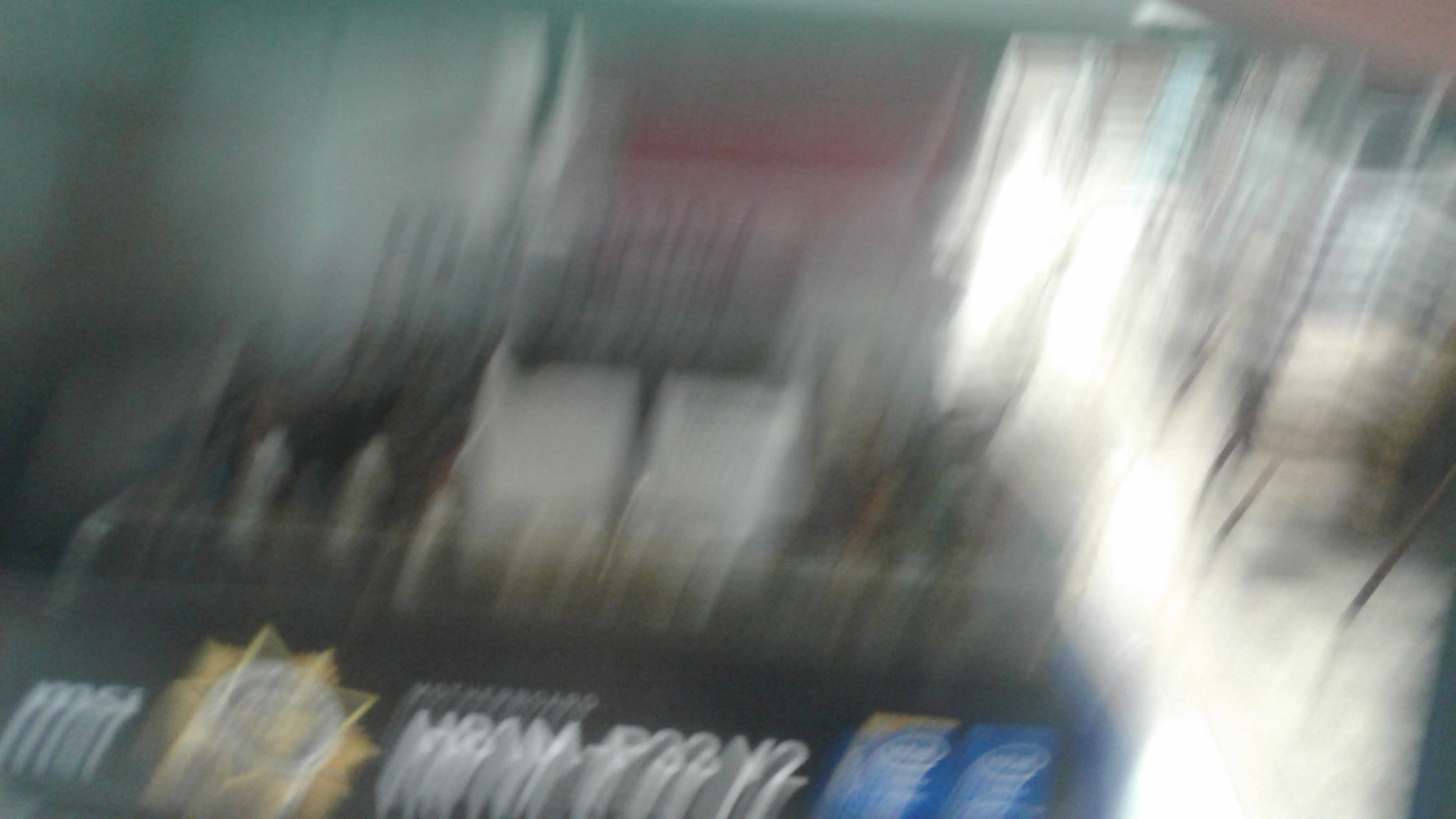The image depicts a fast action shot that is quite blurry, making it hard to discern finer details. At the forefront, a bright white light prominently illuminates the scene. A black rectangle, resembling a computer chip, takes center stage with the inscription "H81M-P33V2" boldly marked in red. Below it, two Intel stickers in blue catch the eye. To the left, the brand "MSI" is visible.

In the background, the framing suggests that this might be a bustling new building, possibly a modern police precinct, hinted at by numerous surrounding towers. There's a splash of red that stretches all the way to the background, complementing patches of white scattered throughout. Adding a touch of nature to the scene, green plants are partially visible, likely on display. Overall, the photograph captures a dynamic and blurry scene, giving an impression of rapid movement and a lively environment.